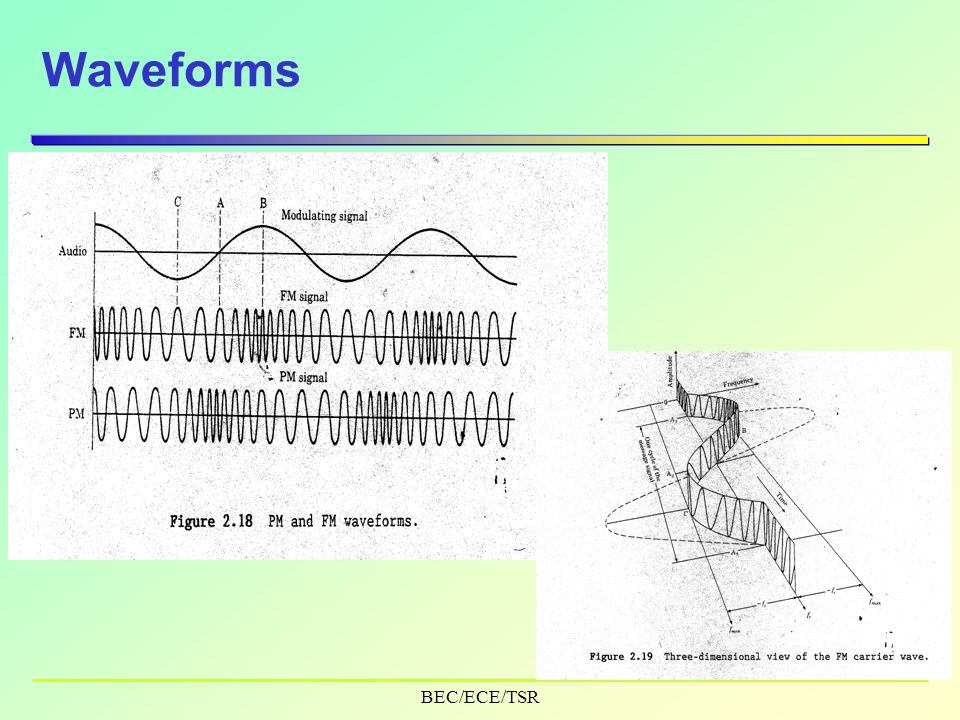The image features a presentation slide with the title "Waveforms" in dark blue lettering at the top left corner. Below the title is a gradient line that transitions from navy blue on the left to yellow on the right, passing through shades of purple near the middle. The background of the slide consists of a gradient from lime green in the upper left corner to yellow in the lower right corner. At the bottom, labels read "BEC/ECE/TSR."

The slide contains two diagrams: the first diagram (Figure 2.18) displays PM and FM waveforms, with three stacked graphs labeled "Audio" (showing a modulating signal with markings C, A, and B), "FM signal," and "PM signal." The diagrams resemble scans from a book and have a somewhat dusty appearance, suggesting low photo printing quality. 

The second diagram (Figure 2.19) presents a three-dimensional view of the PM carrier wave, with its complex waveform depicted in a dynamic, wavy style that moves from front to back, resembling a snake with its curves.